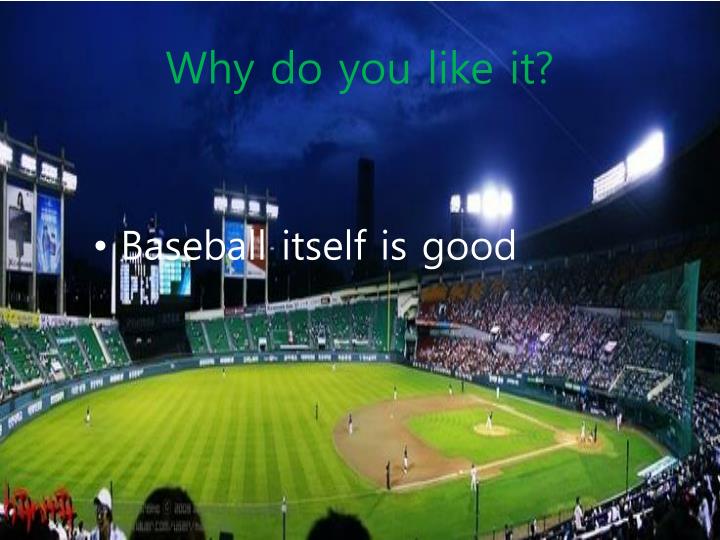The photograph showcases a detailed view of an outdoor baseball stadium taken from a high vantage point, highlighting the entire field and surrounding elements. At the heart of the image lies the neatly manicured, green grass diamond fan-shaped field, predominantly surrounded by a contrast of tan dirt, especially evident on the right side where the home plate is located. Clear white lines demarcate the bases, the pitcher's mound, and the batter's boxes. 

Encircling the field, an array of tiered green seats extends upward, filled with spectators appearing as tiny dots, indicating a large, engaged crowd. The stadium is adorned with numerous signs and advertisements, adding vibrant colors that blend with the overall scene—specifically shades of blue, green, white, red, and brown. Looming overhead, towering floodlights brightly illuminate the field, revealing that the game is taking place under a nighttime sky, which displays patches of whitish areas.

In the top part of the image, green text spells out, "Why do you like it?" with an emphasis on the capitalized 'W' and a question mark, suggesting an interactive or reflective element to the scene. The composition also hints at a digital render, possibly signifying a blend of real and virtual, reminiscent of a video game or a digital screen interpretation. Notably, towards the right, behind the home plate, a large green net is visible, designed to protect the audience from stray baseballs, while a more concentrated group of spectators is visible in the lower left-hand side, directing their attention towards the field.